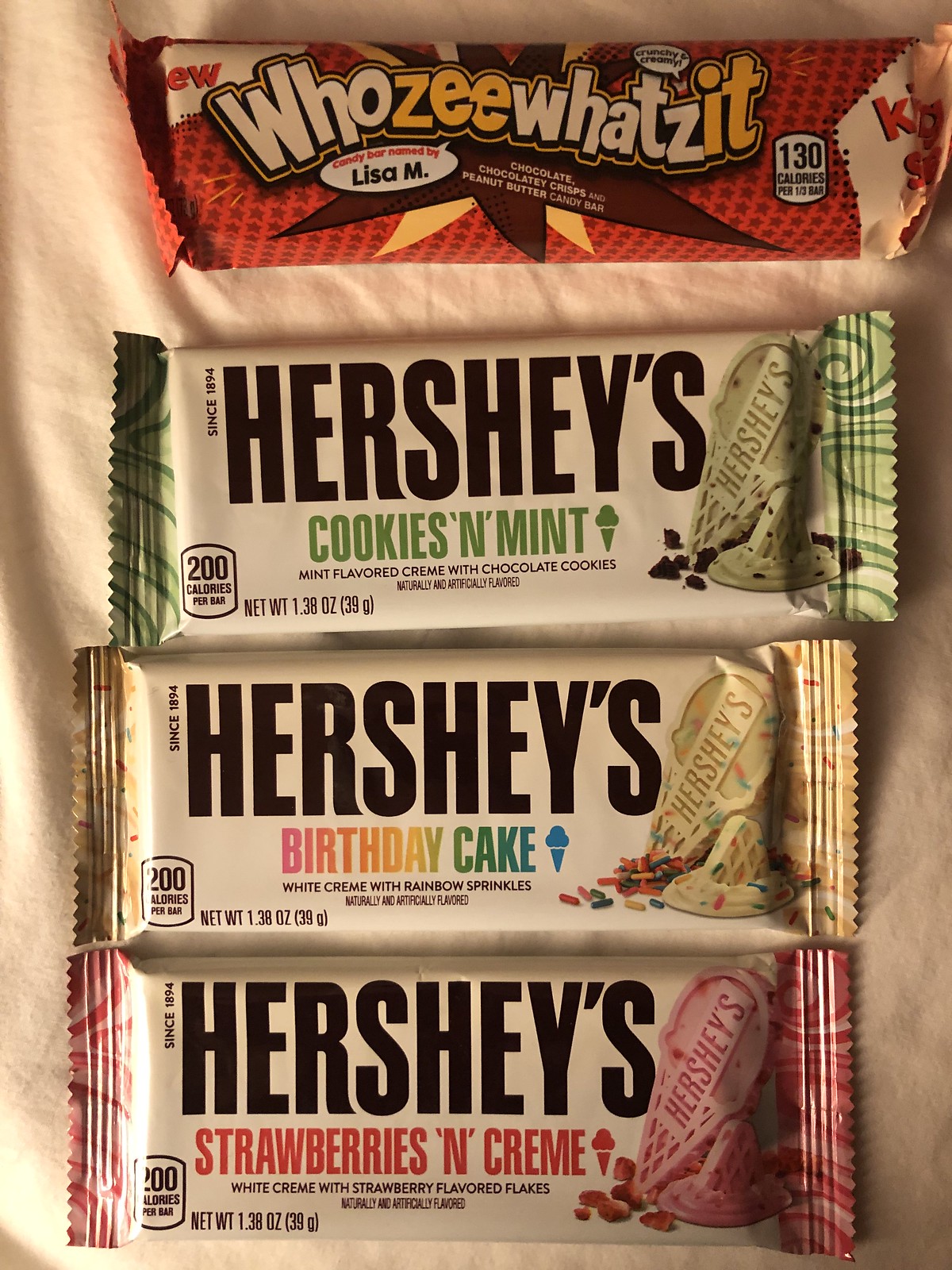This is a top-down photograph of four candy bars neatly arranged in a vertical column on a white fabric surface. All but the top candy bar are Hershey's brand. The top candy bar is a "Who's-E What's-It" in dark red packaging adorned with little stars, featuring bold block letters spelling out the name. This bar is filled with chocolate, chocolate crisps, and peanut butter, marked with 130 calories. 

The second candy bar down is a Hershey's Cookies and Mint bar, identifiable by its flat, rectangular shape and a white wrapper accented with mint green on both edges. The Hershey's brand is prominently displayed in large black letters, with "Cookies and Mint" written in a minty green font.

Next is the Hershey's Birthday Cake bar, which sports a white cream base speckled with rainbow sprinkles. The left and right edges of the wrapper have a frosting-like beige color with sprinkles. The words "Birthday Cake" are written in a gradient rainbow effect, reflecting the festive nature of the flavor.

The bottom bar is a Hershey's Strawberries and Cream, wrapped in a white package with pink edges. The graphic design includes images of strawberries, enhancing the flavor's visual appeal. Like the Birthday Cake and Cookies and Mint bars, this one also features the Hershey's branding prominently. 

All three Hershey's bars have images of the candies they contain and are marked with 200 calories each, carrying a net weight of 1.38 ounces. The photograph is illuminated from the left, adding depth and highlighting the textures of the fabric and candy wrappers.